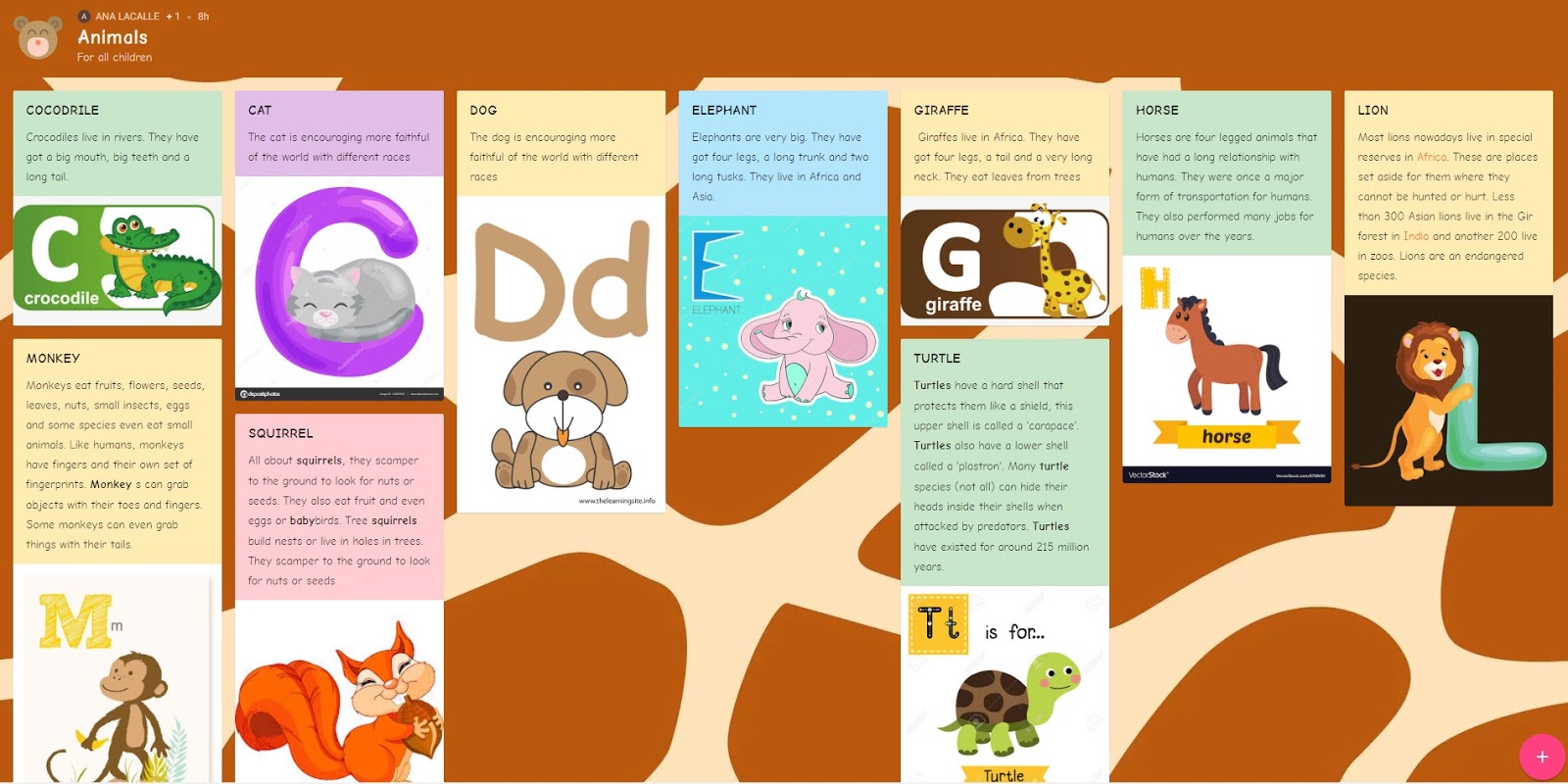This colorful educational poster is designed for children to learn about animals and the alphabet in an engaging way. Titled "Animals," with a subtle subtitle "For All Children," it features large, playful illustrations and fonts that make the learning experience enjoyable for young minds. 

At the top, a prominent bear icon is accompanied by the name "Anakali." The poster is divided into several vertical panels, each focusing on a different animal corresponding to a specific letter of the alphabet. Each panel includes a cute illustration of the animal, the letter it represents, and a brief, child-friendly description.

For instance, the panel for "C" features a green cartoon crocodile with the description: "Lives in a river and has a big mouth." Similarly, the panel for "C" includes a cat illustration with a note that cats symbolize faithfulness, a quality encouraged in school settings.

The poster employs bright colors and animations to captivate children's attention, making learning about animals and letters both informative and fun.